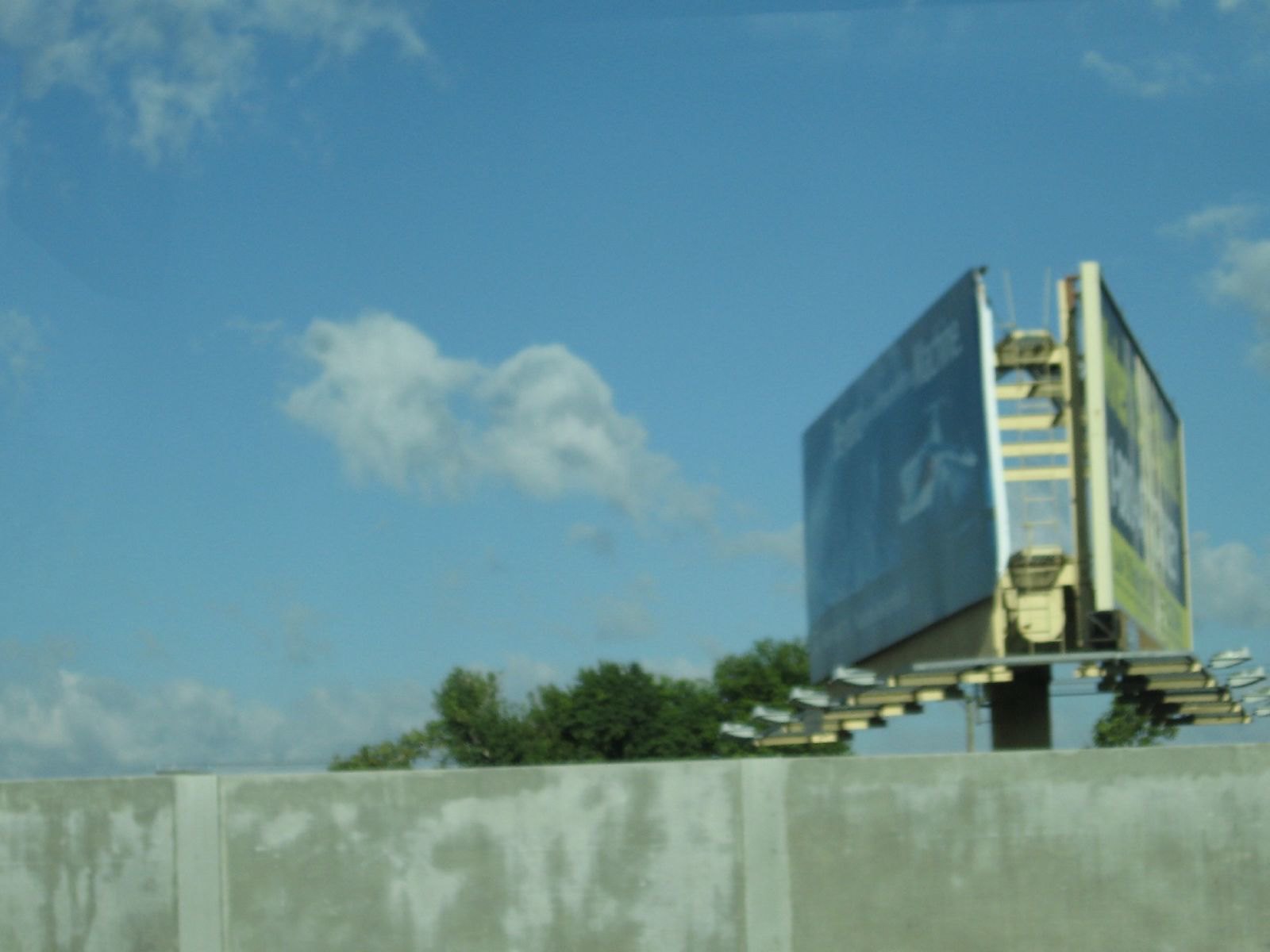This outdoor photograph showcases the side of a multi-colored concrete wall at the bottom. The wall is characterized by patches of white paint, areas tinged with green, and accented with vertical white lines creating an interesting texture. Rising from behind this wall on the right side is a black pole supporting two billboards. Only the sides of these billboards are visible, marked by distinctive white edges. 

At the top of the pole is a yellow-white, smaller square structure, layered underneath a second, similar square. Thick horizontal pieces of white metal stretch between the billboards, providing structural support. Below these billboards, several gray metal poles extend outward, each ending with a streetlight head aimed to illuminate the signage.

To the left of the billboards, greenery peeks into the frame, with the tops of some verdant trees making an appearance. The background is capped off by a vivid blue sky filled with fluffy white clouds, adding a serene ambiance to the overall scene.